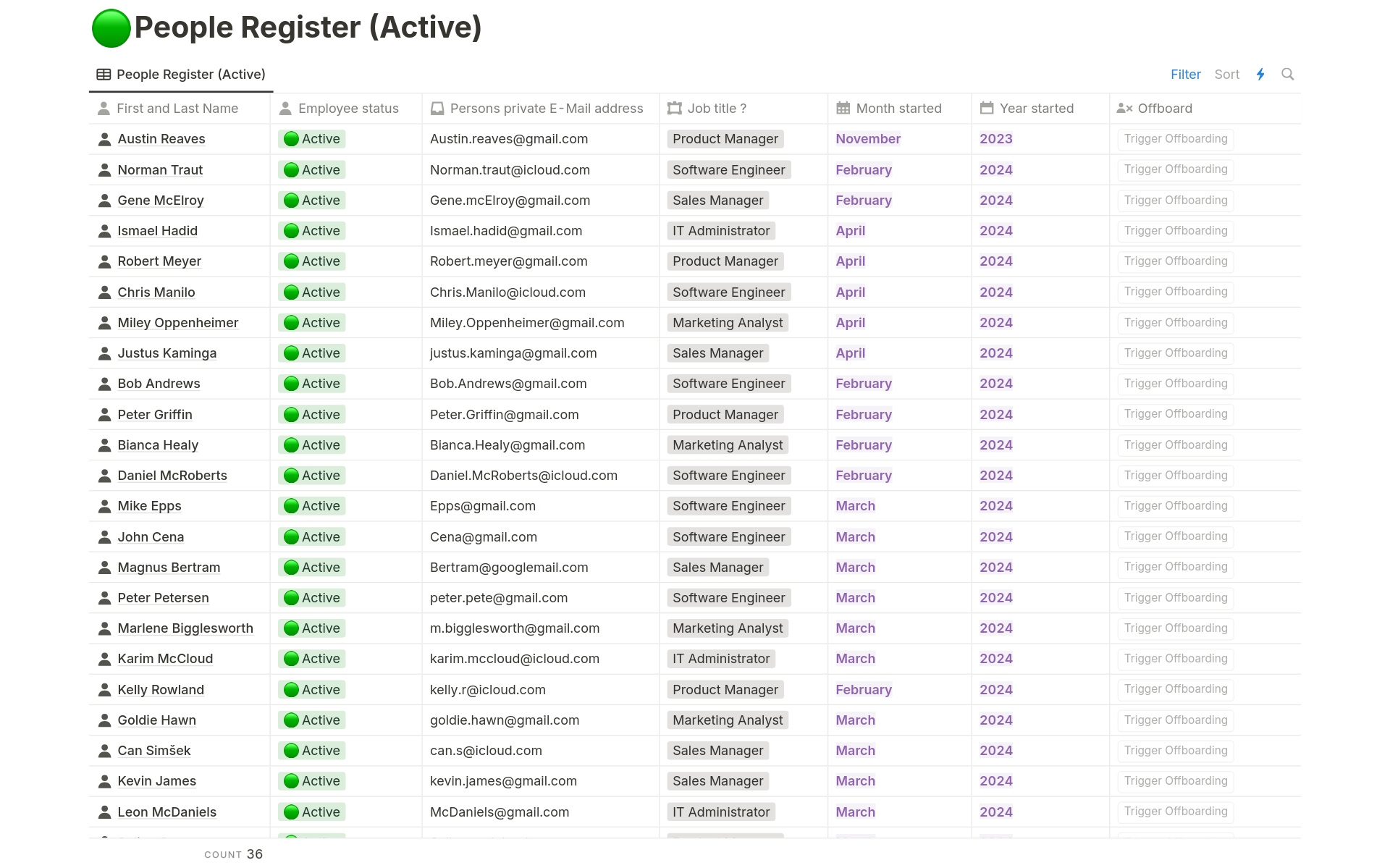In the top left corner of the image, there is a prominent green circle with the label "People Register (Active)" beside it. Beneath this header, the term "People Register (Active)" appears again, emphasizing the section's title. The register categorizes information into sections: First and Last Name, Employee Status, Person's Private Email Addresses, Job Title, Month Started, Year Started, and Off Board.

Under the "First and Last Name" category, a list of several names is displayed: Austin Reeves, Nerman Trout, Gene McCoy, Robert Meyer, Chris Manilla, Bob Andrews, Peter Griffin, Bianca Healy, John Cena, Mike Epps, Karen McLeod, Kelly Rowland, Kevin James, and Leon McDaniels.

For "Employee Status," each individual has a green circle next to their name, indicating their status as "Active."

The "Person's Private Email Addresses" category lists the private email addresses of each employee. 

The "Job Title" section features titles within gray rectangles, such as Product Managers, Sales Managers, IT Administrators, and more.

Under the "Month Started" category, various months are listed in purple.

The "Year Started" section lists the years in purple, ranging from 2023 to 2024.

Lastly, under the "Off Board" category, there is an option labeled "Trigger Off Boarding" for each employee.